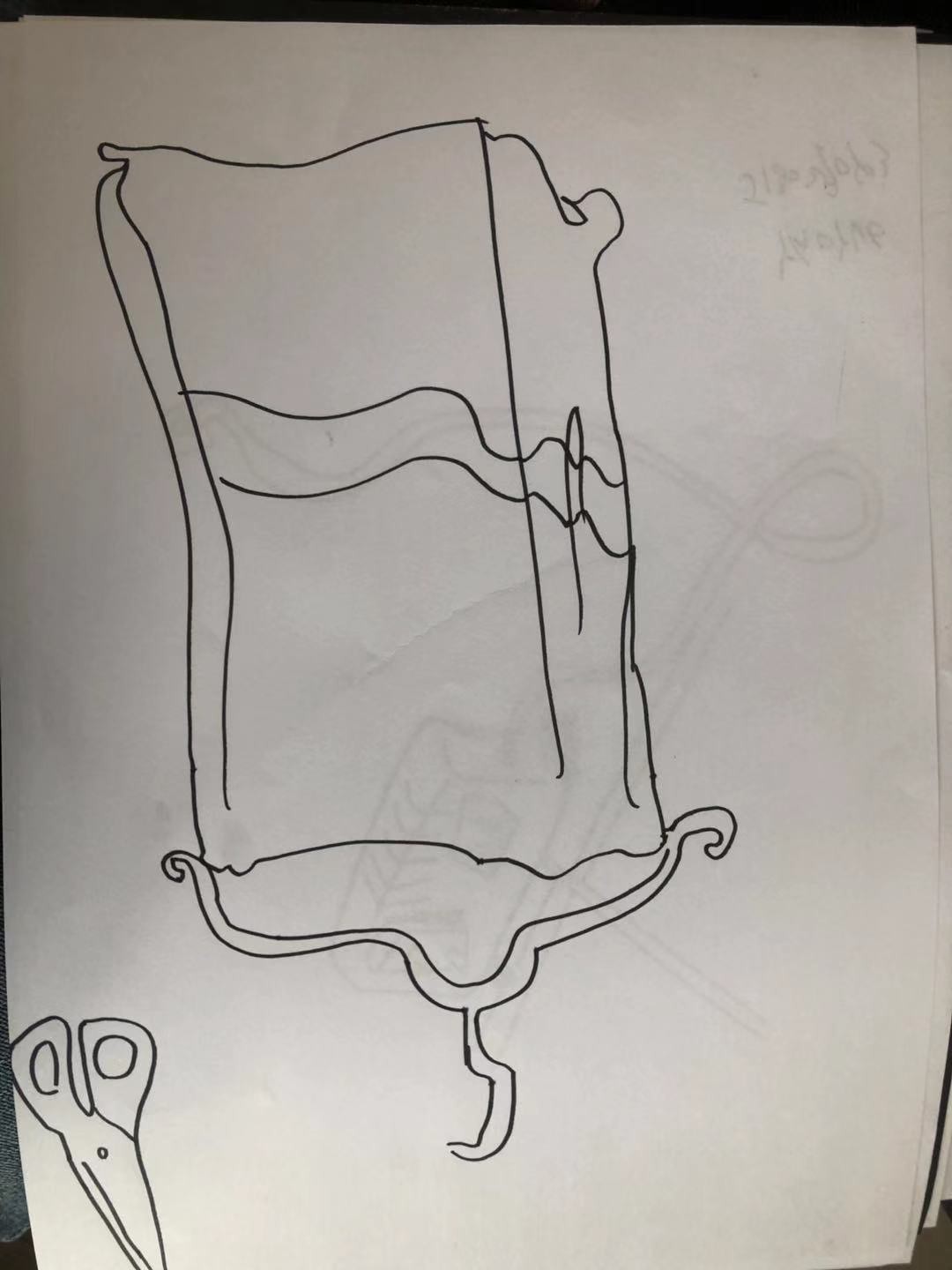This image is a hand-drawn illustration rendered with markers. In the bottom corner, a detailed depiction of a pair of scissors is prominently featured. Adjacent to the scissors, an inverted clothes hanger or a piece of clothing is discernible, adding a whimsical element to the composition. The bottom corner of the drawing also contains some handwritten text, although it is partially unclear and tough to read.

Beneath the main drawing, the paper has additional outlines or images that are likely intended for coloring or further detailing. The background outside the paper suggests that the image might have been taken in a casual setting, possibly in an office or on a couch, as indicated by the presence of what appears to be a cushion. The paper itself is pristine white, resembling standard printer paper, and occupies almost the entirety of the frame.